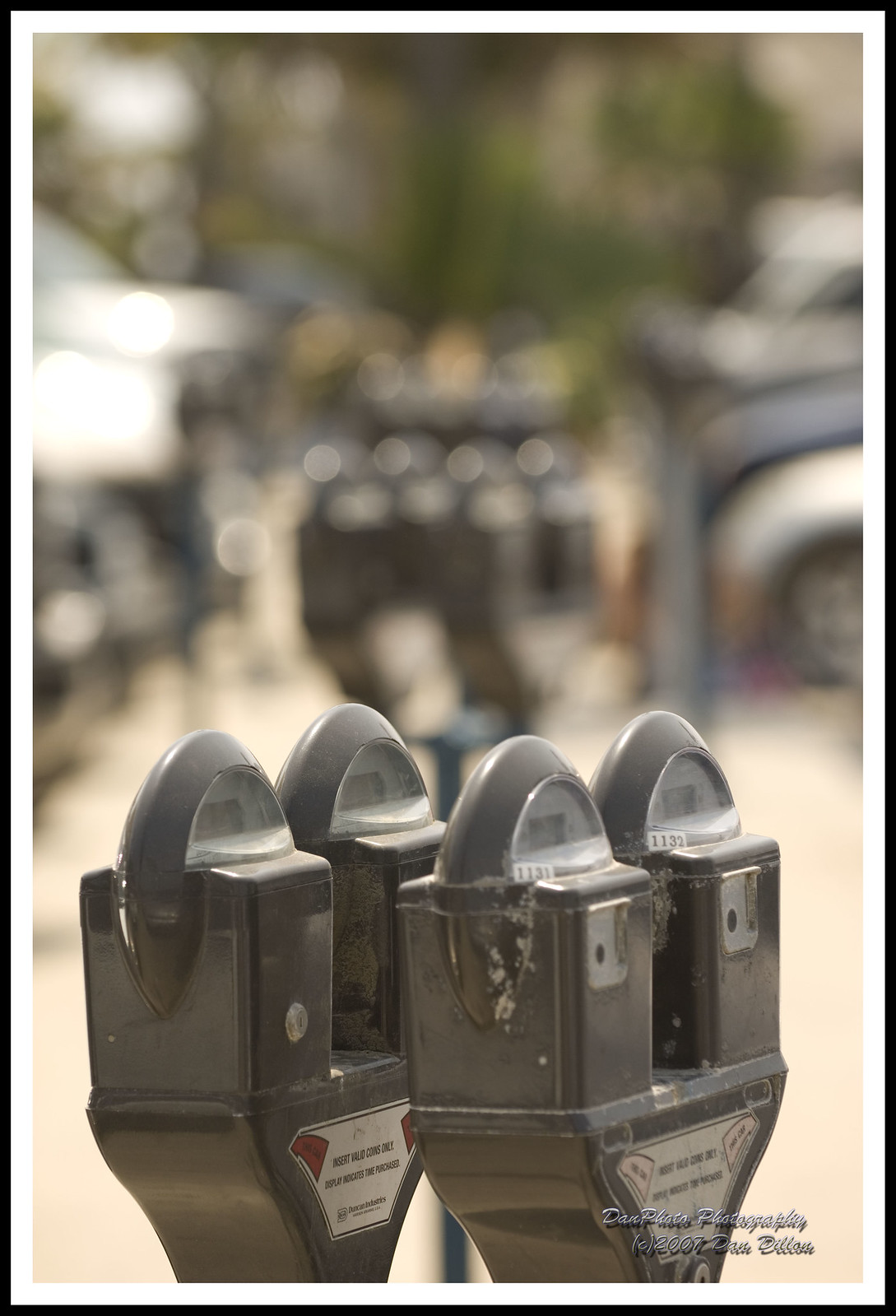The image presents a vertical orientation, approximately one and a half to two times taller than it is wide, depicting a curb or parking median flanked by blurry cars on both sides. On this cement area between parking spaces, there are two distinct pairs of parking meters in the foreground, forming a Y-shaped structure and topped with dome-like caps. Each dark grayish black meter has a silver plaque and displays remaining time within its dome and exhibits some chipped paint, likely from frequent contact.

Further in the background, another set of two parking meters is visible, though blurred, along with several cars—two discernible on the right and three on the left, with a white car and its tire particularly noticeable on the right side. The scene is sunlit, creating a glow on the car hoods. Additionally, there is some greenery visible above the central parking meters, suggesting the presence of trees or plants. The image also includes small, unreadable text on the bottom right-hand side, and the overall background maintains a significant level of blur.